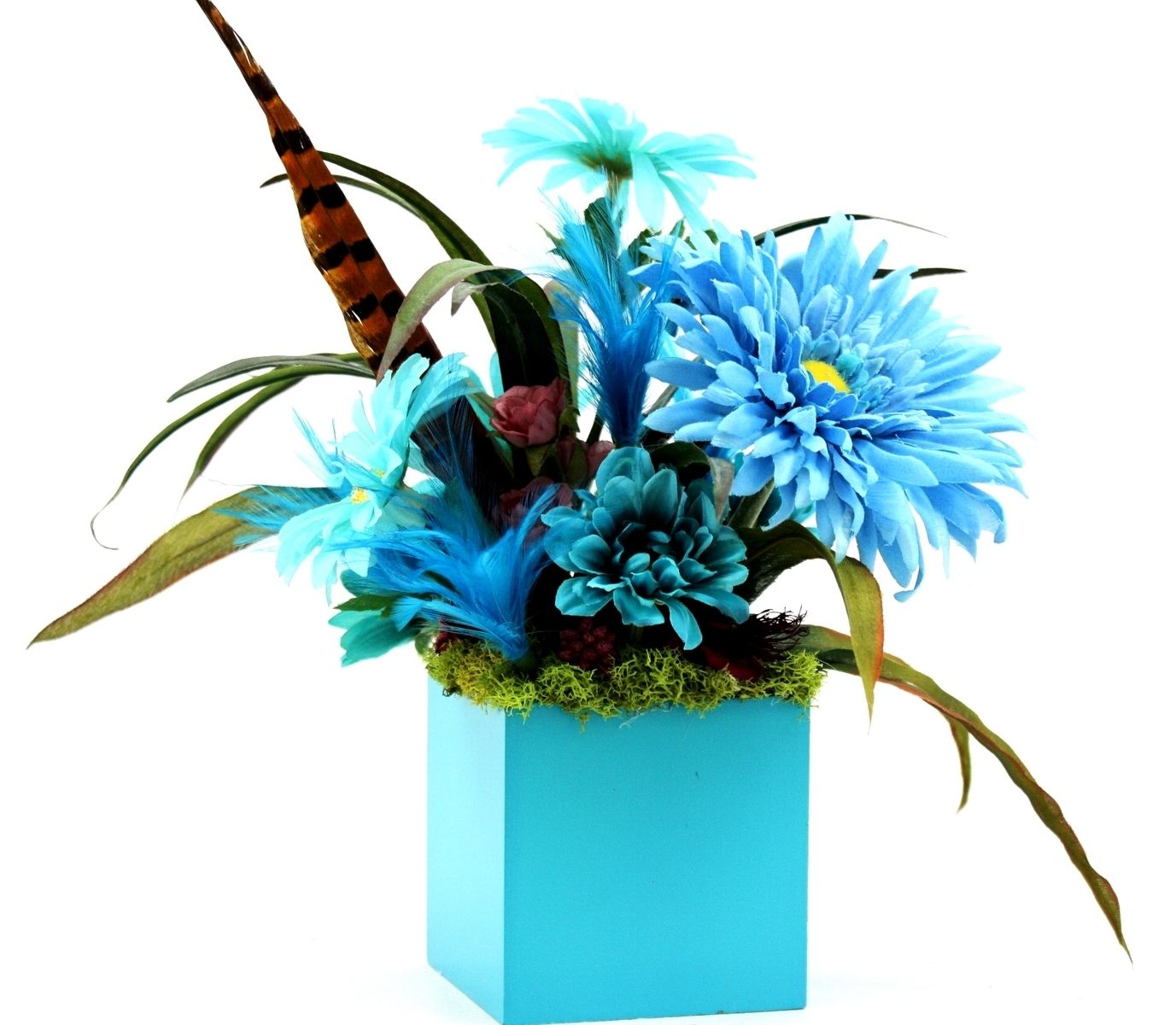The image showcases a meticulously crafted painting of a lush, floral arrangement set in a blue, cube-shaped planter. The planter appears vividly in the foreground with no evident border, set against a stark white background that provides contrast and emphasizes the colors within the artwork. The planter has a lit side, highlighting its square form. The base of the arrangement is lined with green moss, from which emerges a diverse bouquet. Dominating the composition are various hues of blue flowers, some with translucent petals that reveal the leaves beneath them. In the upper left section, a brown and black feather adds an unexpected texture. Green leaves and grass material further fill out the arrangement. Notably, there is a vibrant blue flower with a yellow center on the right, a smaller blue flower in the center, and a striking red and black leaf extending outward from the left side. The predominant color theme of the artwork is blue, underscored by the blue planter and the five different shades of blue flowers, accented with green foliage, creating a visually harmonious and balanced piece.